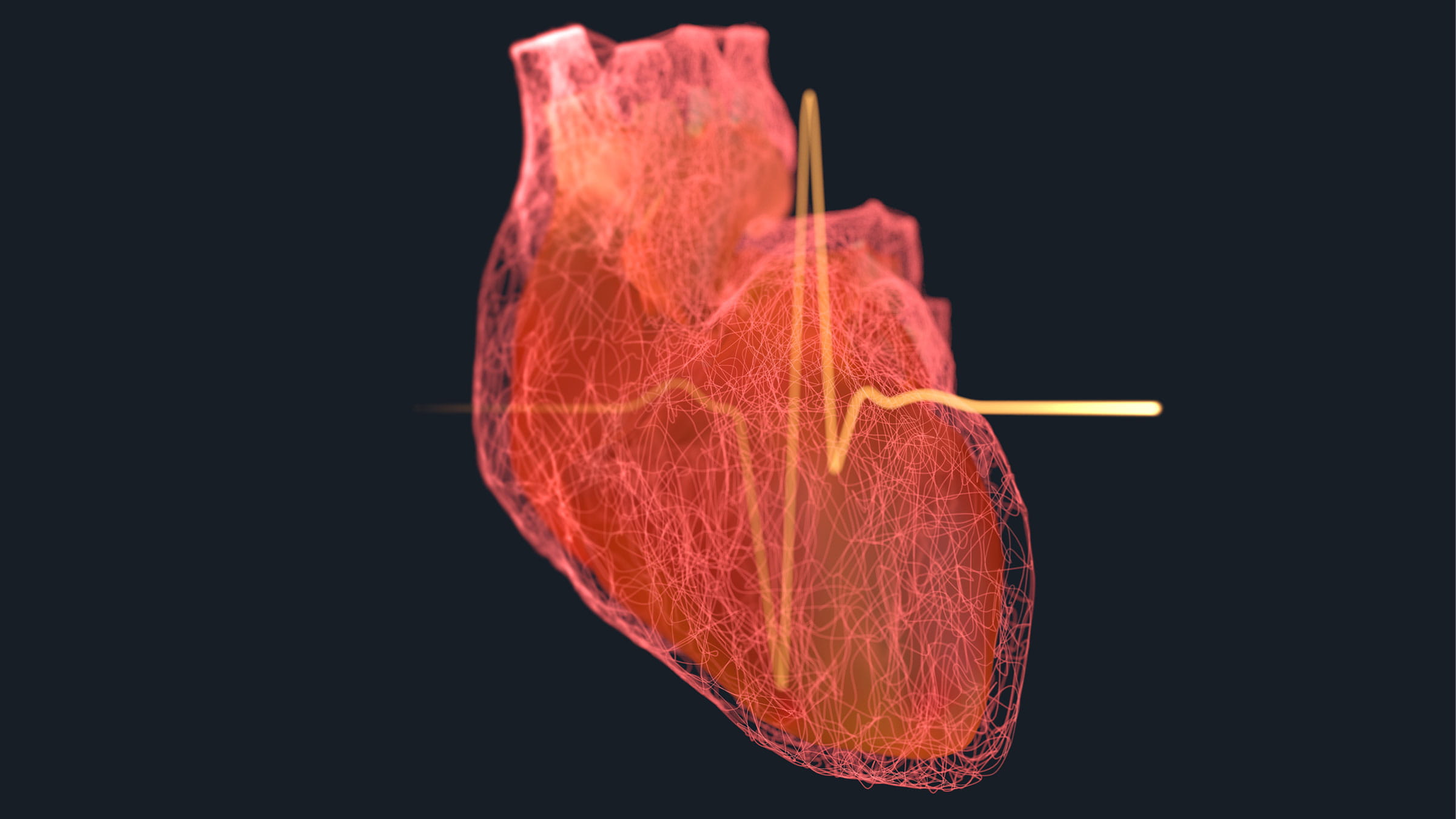The image is a detailed illustration of a human heart rendered in various shades of red and peach, displayed against a plain black background. The heart occupies the center of the image and is viewed from a side profile, giving it a two-dimensional appearance. Fine, lighter red lines representing veins run throughout the heart, with the overall structure outlined in a transparent red and the center appearing in a darker, slightly opaque shade. Superimposed on the heart is a vibrant yellow heart monitor line, depicted as a series of sharp peaks and valleys akin to a heartbeat visual sensor found on medical equipment. This yellow line, which stands out brightly against the black background, further suggests the heart's rhythmic activity, emphasizing that the image is a computer-generated design rather than a real anatomical photograph.